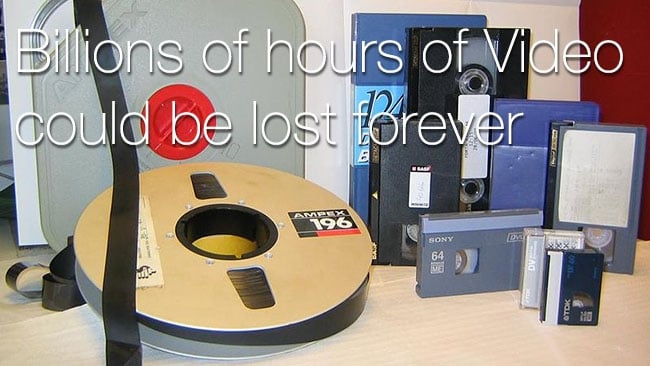The image presents a nostalgic collection of various old-style recording media set on a beige, almost pinkish, covered table surface. To the left, a light wood brown and black film reel, labeled "Amprex 196," is accompanied by some loose film and a gray case behind it. On the right side, an array of cassettes is displayed, arranged by size. Closest to the front are smaller cassettes, including brands like TDK and Sony, and a DV cassette. Behind these, larger media like VHS and Betamax cassettes create a gradient of ascending sizes. In the very back, a blue and purple book peeks out amongst the tapes. The background text, in white, emphasizes the urgency to preserve these memories with the message: "Billions of hours of video could be lost forever."